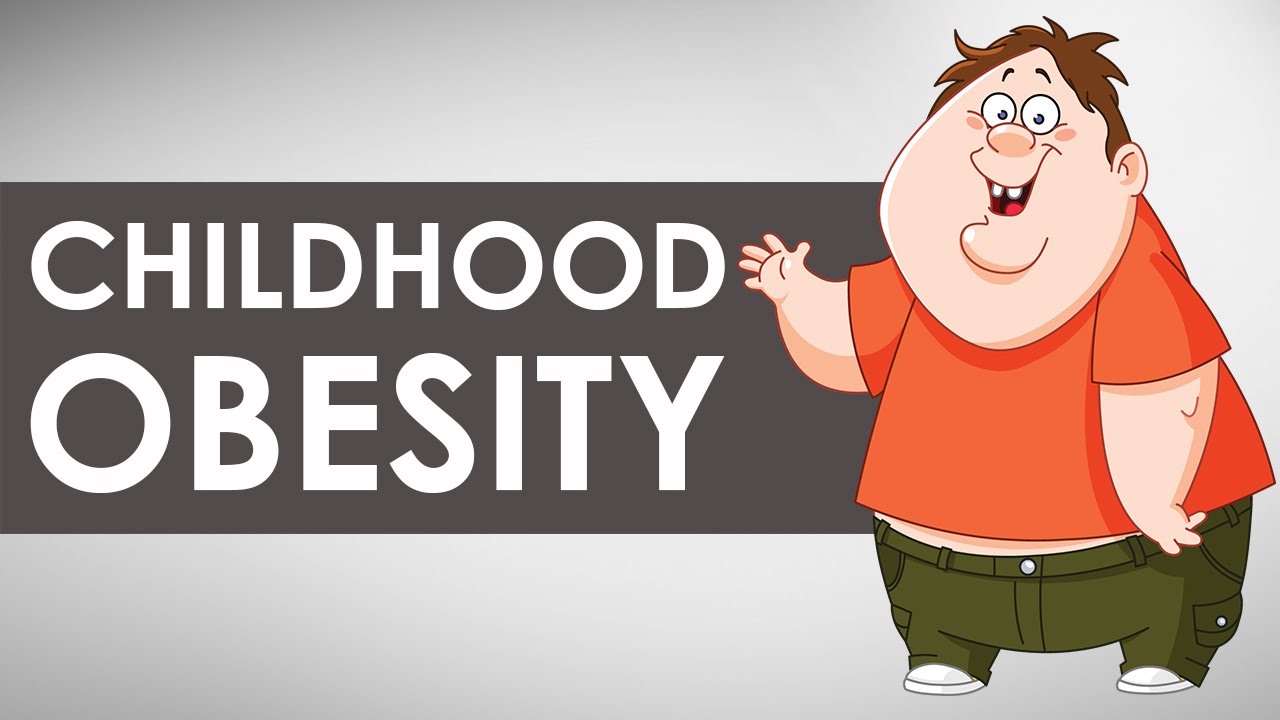The image is a detailed clip art graphic of a smiling, overweight boy with short brown hair, two buck teeth, and a large round face with no neck. He is wearing an orange t-shirt, dark green pants, and white shoes. The boy is depicted waving. To the left of him, there is a dark gray rectangle featuring the white text "childhood obesity." The entire scene is set against a light gray background. The boy's cheerful expression contrasts with the serious message conveyed by the text.